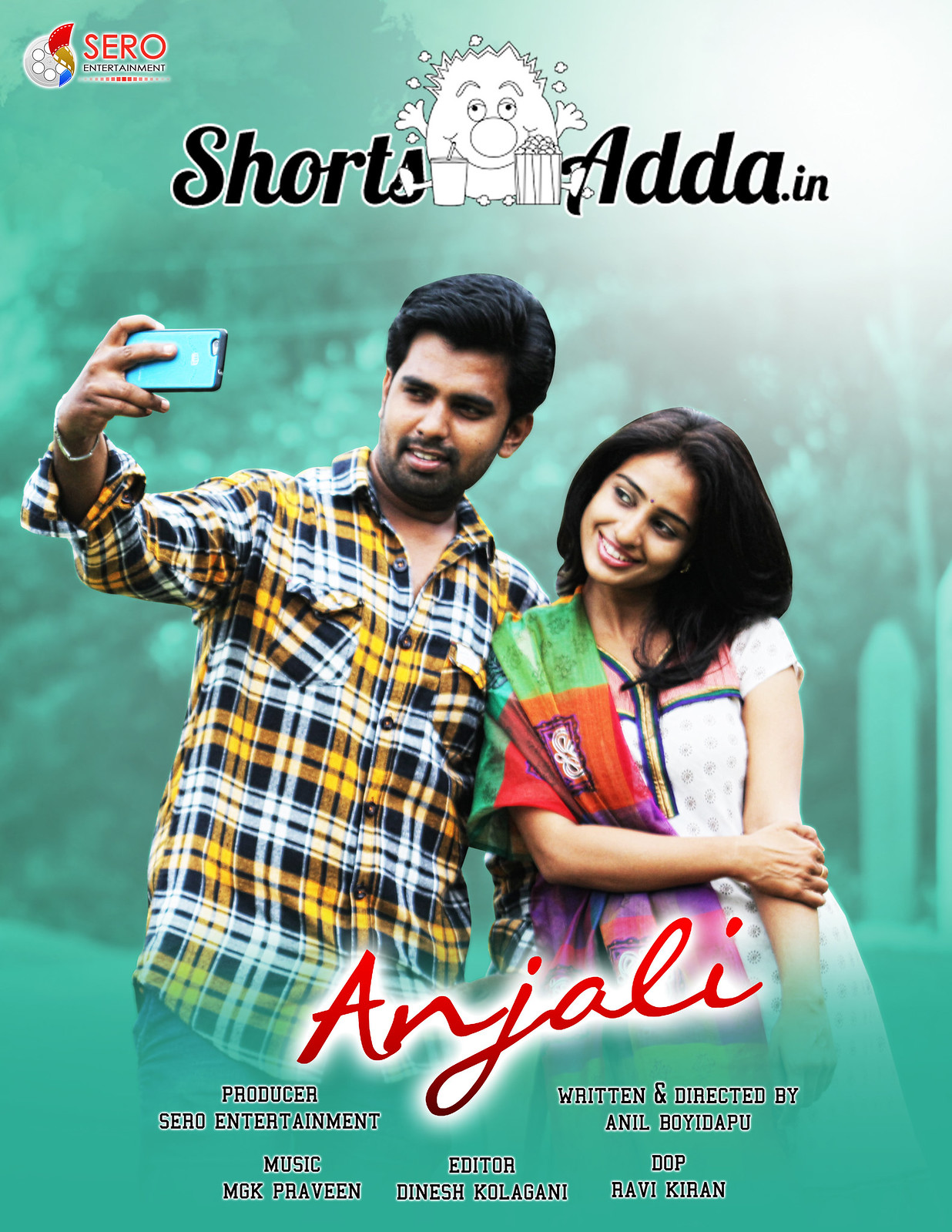The poster for the short film titled "Anjali" features a vividly colored green and blue background with a slightly blurred garden-like image. At the top, it reads "Shorts Adda" with an accompanying logo of an animated white-faced character munching on popcorn and sipping soda. Dominating the middle of the poster are the lead characters, a young man and woman, likely of Indian descent, capturing a selfie. The man, positioned on the left, wears a yellow, black, and white striped plaid shirt and has dark, slicked-back hair, holding the camera sideways. The woman on his right, who has a big smile and a bindi on her forehead, is clad in a white dress with pink accents and a multicolored shawl featuring green, orange, and purple patterns. In bold red cursive at the bottom, the title "Anjali" is prominently displayed. The credits, listed underneath, reveal that the film is produced by Cero Entertainment, written and directed by Anil Bhadidapu, with music by MGK Praveen, editing by Dinesh Kolagani, and cinematography by Ravi Kiran.